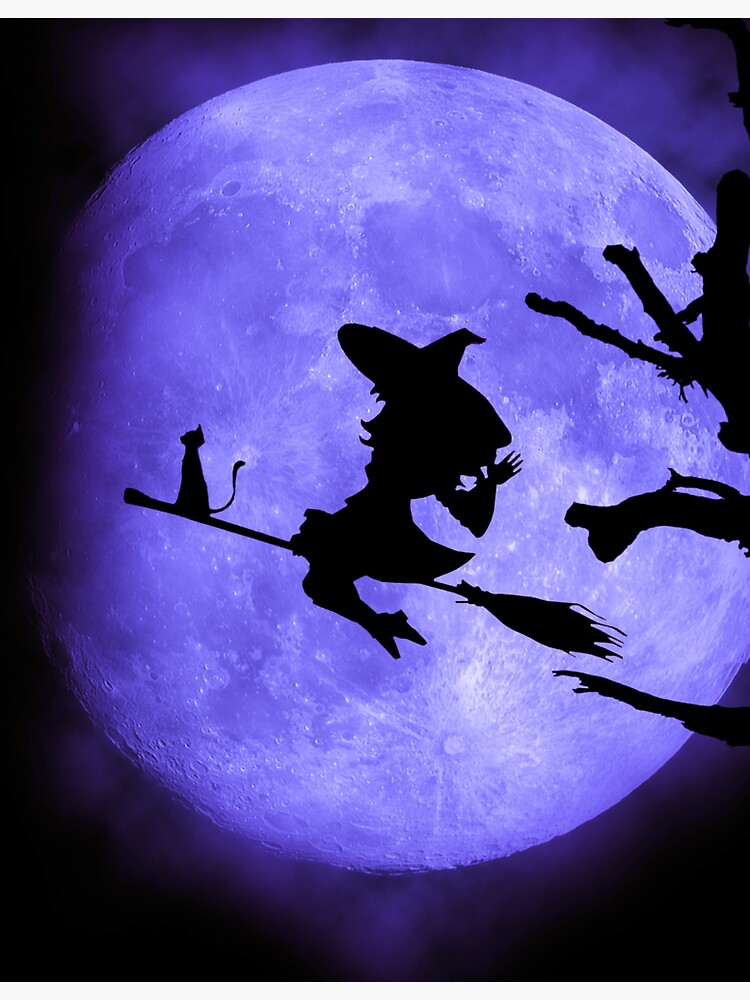In this fantasy art illustration, a large, purple-hued moon dominates the background with darker purple craters providing depth. The moon is set against a nearly black sky. At the center of the moon's glow is the black silhouette of a witch riding a broomstick, heading towards the left side of the image. Her broom is pointed to the right, and she is waving with a bent knee, wearing a large, pointed hat. Accompanying her on the far end of the broomstick, to the left, is a cat, also depicted as a solid black silhouette. Completing the scene, the right side of the image features the leafless, gnarled black silhouettes of tree branches, adding to the whimsical, eerie atmosphere.